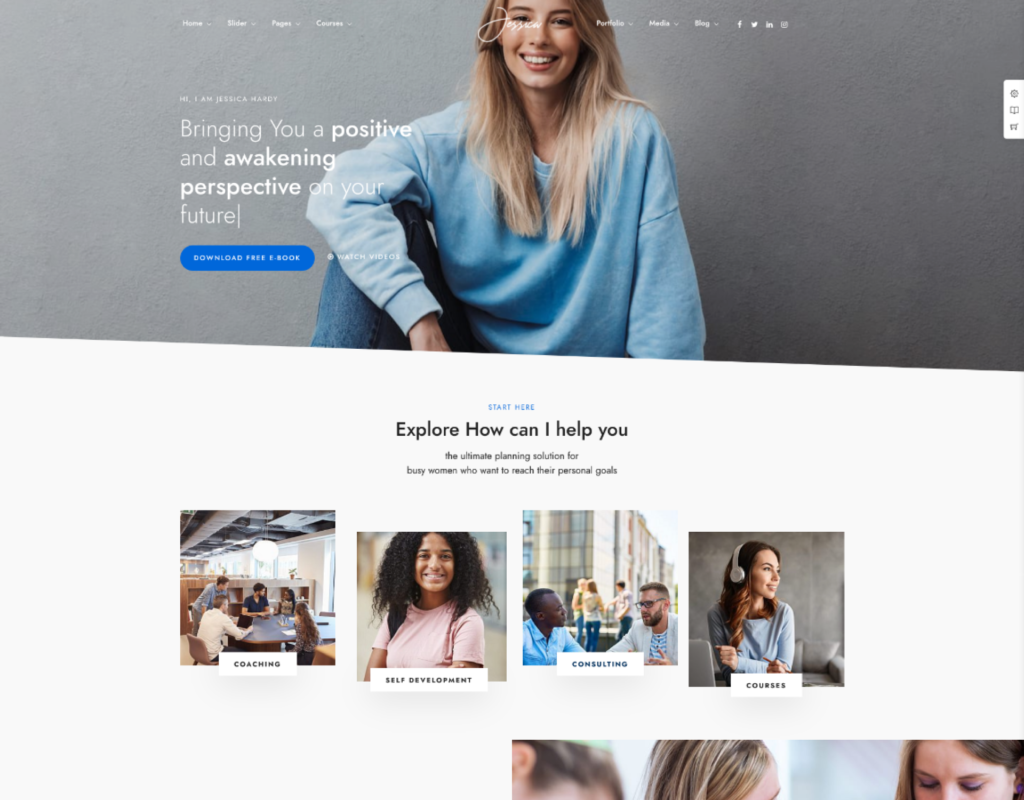Screenshot of a website featuring a headshot of Jessica Hardy, a blonde woman smiling and wearing a blue long-sleeve sweater, set against a gray background. The website's top navigation, although slightly out of focus, includes tabs such as "Home," "Pages," "Portfolio," and "Blog." In the center, "Jessica" is prominently written in cursive font. Below, a message reads, "Hi, I am Jessica Hardy, bringing you a positive and awakening perspective on your future," with a blue button for downloading a free eBook. Lower down, the text on a white background invites visitors with "Start here. Explore how I can help you. The ultimate planning solution for busy women who want to reach their personal goals." It lists services like "Coaching," "Self-development," "Consulting," and "Courses," each accompanied by stock images of people engaging in various activities. In the bottom right corner, there's a partially visible photo of individuals, but the details are unclear.